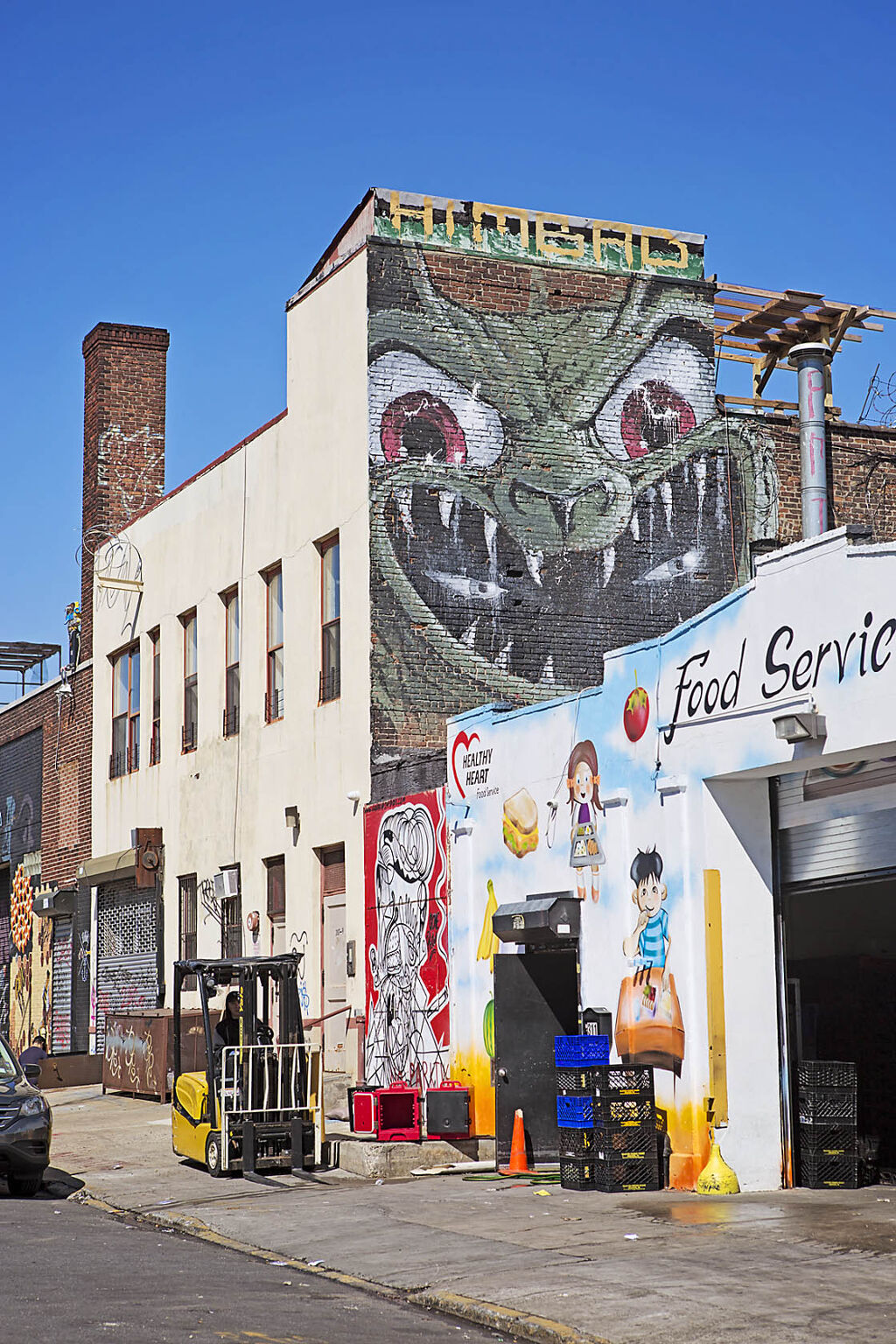The image captures an urban back street scene featuring a collection of interconnected industrial buildings adorned with vibrant murals. The primary focal point is a white building with a mural depicting a bright blue sky filled with images of children and assorted snacks, likely indicating its role in local school lunch services. The mural prominently displays the words "food service" along with "heart healthy." This building is juxtaposed against a gritty cityscape featuring a dirty cement sidewalk littered with red plastic crates.

In the center of the image is a towering brick building with a striking, eerie mural at the top. This artwork features a ghastly goblin-like creature with sharp, white teeth and red, piercing eyes. The word "H-I-M-B-A-D" is scrawled above this grotesque figure. Below this menacing mural are additional graffiti and murals, including bright depictions of apples and bananas that contrast sharply with the monstrous figure above.

The urban street scene includes practical elements such as a yellow forklift positioned on the sidewalk, and a black car either parked or in motion. The sky above is a clear, bright blue, enhancing the contrast of the colorful and varied artworks against the industrial backdrop, completing the snapshot of lively urban art amid functional city infrastructure.